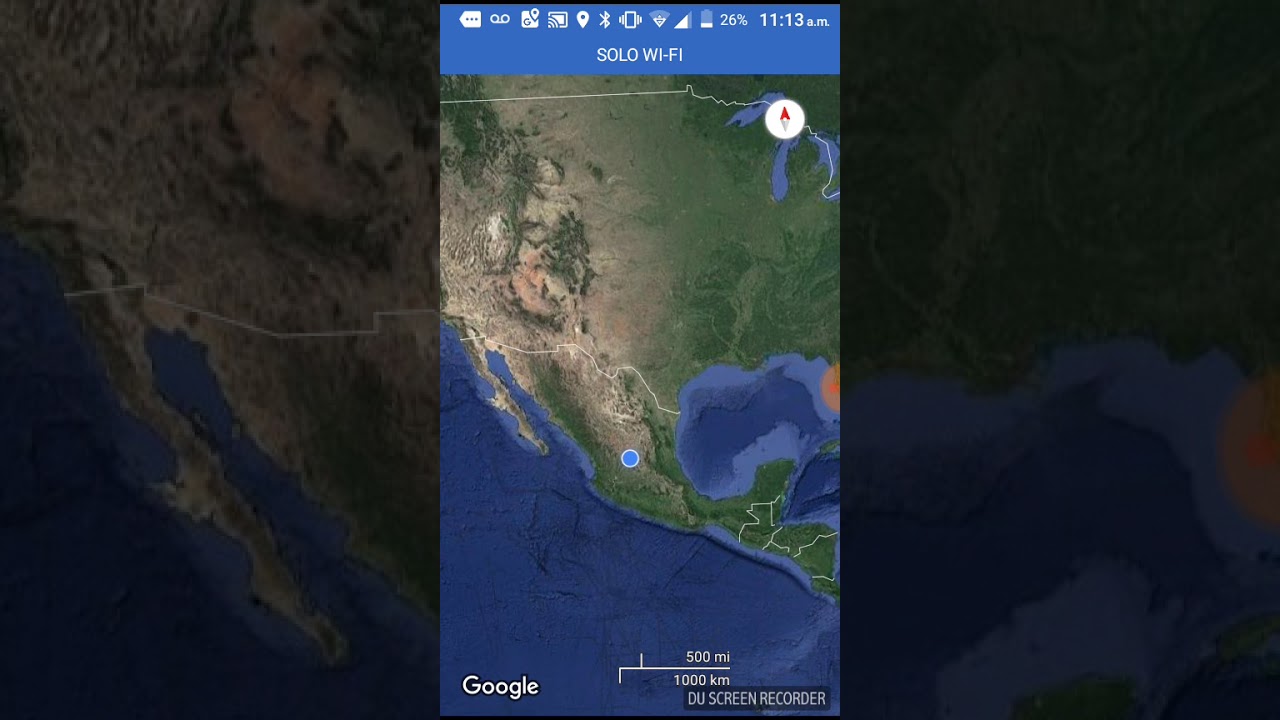This image is a screenshot from a mobile device displaying the Google Maps application. The map is focused on the country of Mexico, with a prominent blue dot marking a location in the central region of Mexico. The image also includes a variety of status icons at the top, indicating the time as 11:13 a.m., a battery level of 26%, and active connections including Wi-Fi, cellular service, Bluetooth, location, and casting. Additionally, a voicemail notification is visible. The bottom left corner of the screenshot features the Google logo, and to its right is an annotation indicating the use of DU Screen Recorder. The map view subtly includes the southern United States on the left and right peripheries, though these areas are dim and less discernable. The screenshot is titled "Solo Wi-Fi," suggesting the map is currently using a Wi-Fi connection. The overall ambiance of the image is slightly dark, perhaps indicating the device’s dimmed screen settings.